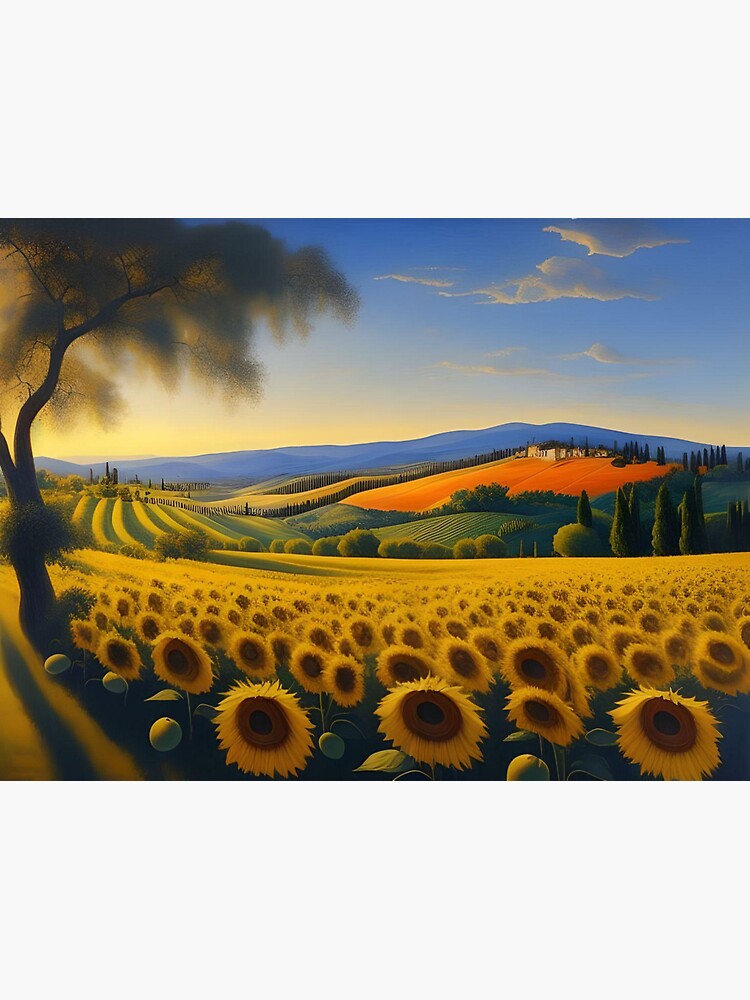This illustration presents a beautifully detailed landscape dominated by vast fields of vibrant sunflowers stretching extensively from the right to the left, primarily occupying the bottom section. The sunflowers, with their faces turned towards the viewer, are vividly yellow, creating a striking contrast against the rest of the scenery. To the left, a tall tree with typical foliage frames the sunflower field. The background reveals a serene countryside with rolling hills and valleys, highlighted by an orange-tinted hill that houses a distant farm or building. The horizon showcases a blue mountain range under a clear blue sky dotted with white clouds. The sky transitions to a warm yellow near the horizon, suggesting a setting sun. This amalgamation of elements, including patches of well-maintained fields with distinct grassy patterns and subtle barricades, creates an expansive and immersive pastoral scene. The entire composition pulls the viewer in, with certain elements artistically stretched to emphasize depth and perspective.